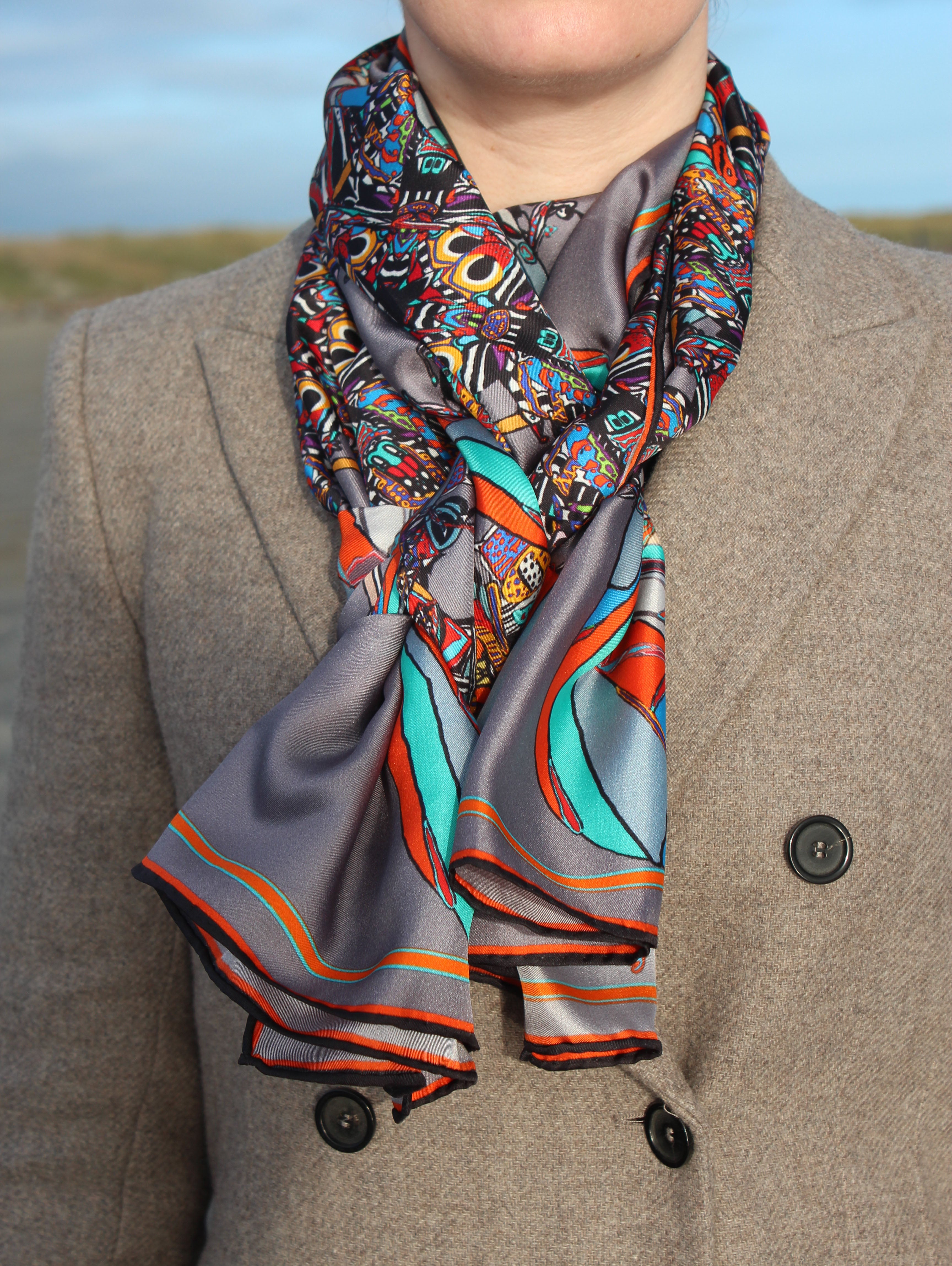The image features a person, likely a man, dressed in a sophisticated gray coat with prominent black plastic buttons. Only the lower part of the person's face, including the chin and part of the neck, is visible, drawing focus primarily to the colorful, intricately designed scarf draped around their neck. The scarf, primarily gray, features an array of vibrant colors such as light blue, turquoise, orange, green, and yellow, along with numerous abstract shapes and patterns, making it appear particularly busy around the neck area while the ends are more muted with solid gray, orange, and black hues. The background suggests an outdoor scene, possibly in the fall, with a green field, some dirt patches, and a sky filled with gray clouds against a pale blue backdrop. This image captures an individual with a keen sense of fashion, highlighting the striking contrast and detailed design of the scarf against the classic, buttoned gray coat.